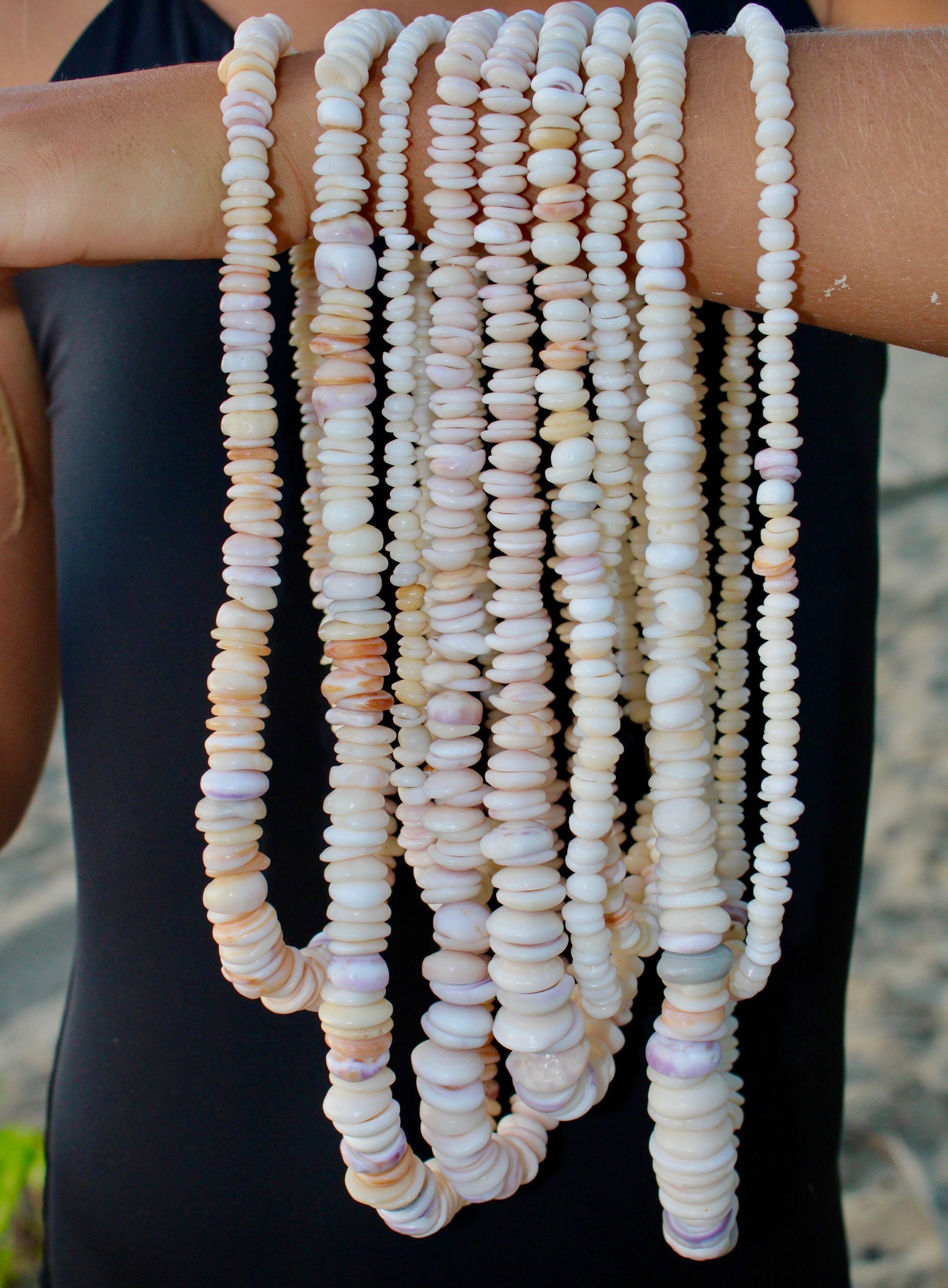In this detailed close-up image, a person with tan skin and wearing a form-fitting black tank top, possibly a bathing suit, is showcasing several necklaces draped across their forearm, with the forearm crossed over their chest. The background is a blurred gray area, adding focus to the subject. The necklaces, predominantly made of round, disk-like objects resembling puka shells, are strung together in various shades of pink, white, tan, and yellow. These shells range in size, with some necklaces extending up to a foot long while others are about five to six inches long. The necklaces, totaling around nine, vary in thickness and the size of the shells, giving a mixed yet harmonious display of what looks like Hawaiian-inspired jewelry.